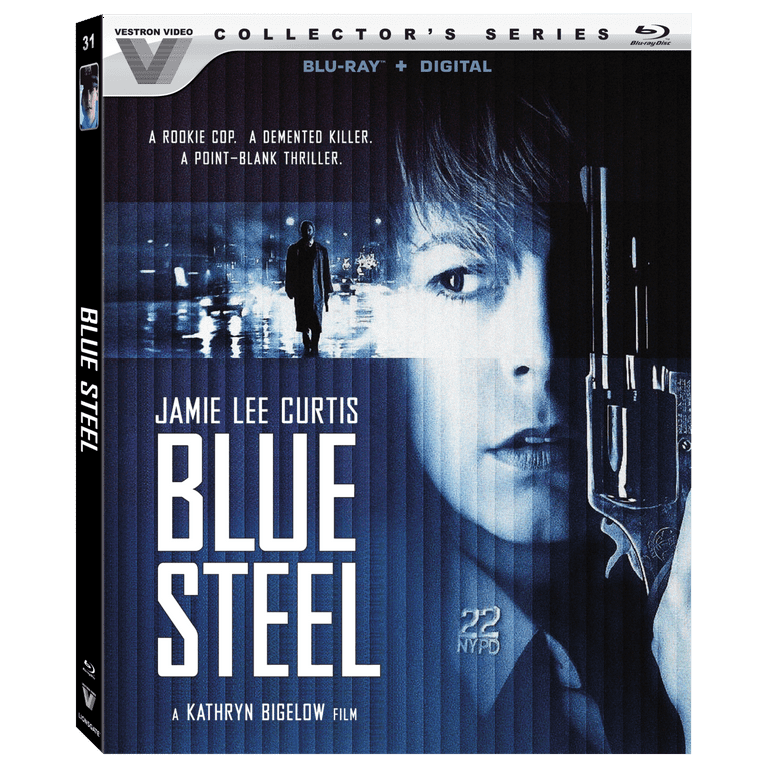This detailed caption captures the shared and emphasized details from the three descriptions:

The image showcases a Blu-ray movie case for the film "Blue Steel," featuring Jamie Lee Curtis prominently on the cover. The overall design of the case uses hues of blue, black, and gray, setting a suspenseful and murky tone. Jamie Lee Curtis is depicted wearing a police uniform with "22" and "NYPD" visible on the collar of her collared shirt. She looks worried, her eyes directed towards her right, while holding a revolver up to her face, partially obscuring it. To the left of her face, there's an indistinct image of a man in a long overcoat walking down a nighttime street towards the camera. The top of the case displays the logo and text "Vestron Video Collector Series," followed by "Blu-ray plus digital." Below this, in white lettering, the text reads, "A rookie cop, a demented killer, a point-blank thriller." The main title prominently features Jamie Lee Curtis's name, the movie title "Blue Steel," and credits Catherine Bigelow as the director. Overall, the cover suggests a suspenseful and potentially violent thriller.